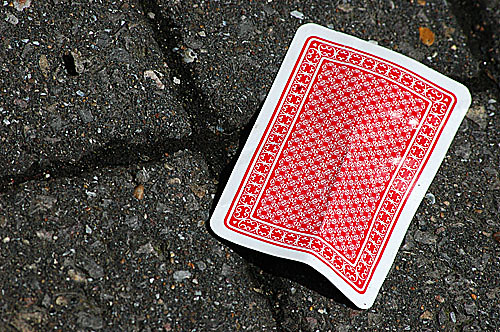The photograph captures an outdoor scene featuring a textured surface composed of square tiles, each separated by dark black grout. The squares are predominantly light black, with specks of rock or dirt scattered across them, adding a rugged texture to the flooring. 

A single playing card is prominently displayed on the tiles, slightly bent down the middle and tented, hinting at previous use or wear. The card's top side features a distinctive design with a thick white border encasing a larger red-and-white patterned rectangle. This pattern includes motifs resembling little clouds and star-shaped columns, framing a central rectangle adorned with a white floral design. The card, slightly tilted to the right, draws attention with its vivid red and white color scheme against the subdued background of the tiled floor.